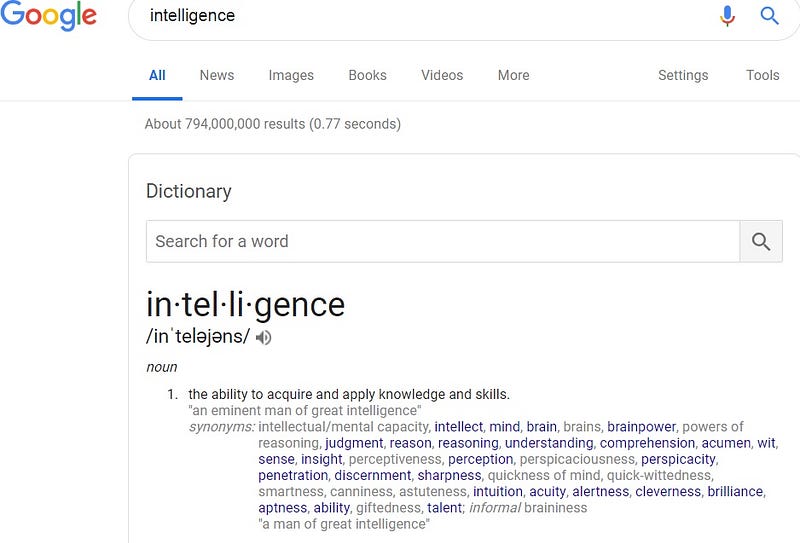The image depicts a Google search results page for the term "intelligence." On the top right of the search bar, there's a blue microphone icon. Below the search bar, the "All" tab is highlighted in blue, with other options like "News," "Images," "Books," "Videos," and "More" displayed in gray. Towards the right, settings and tools options are available.

The search yielded approximately 794 million results in less than a second. Directly beneath the search bar, a dictionary entry for "intelligence" is prominently displayed. This entry includes:

- Phonetic breakdown of the word for pronunciation assistance.
- A speaker icon to hear the correct pronunciation.
- The classification of "intelligence" as a noun.
- The definition: "The ability to acquire and apply knowledge and skills."
- An example sentence in quotes.

Following the definition, a list of synonyms is provided, such as "intellectual," "mental capacity," "intellect," "mind," and "brain," all of which are hyperlinked in blue to allow further exploration.

The webpage maintains a simple, white background, with minimal color emphasizing hyperlinks, the microphone icon, the highlighted tab, and the multicolored Google logo. The visually distinct elements guide the user’s navigation through the search results and resources.